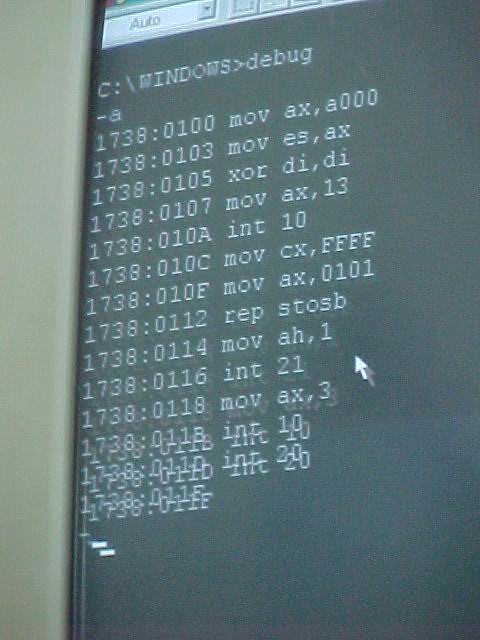This detailed photograph captures a close-up of a computer screen with a dark background, displaying lines of white text. On the left side, the white frame of the computer is visible, and on the right, the screen shows a sequence of commands or code. At the top, an area labeled "auto" with a drop-down button is faintly visible. The code begins with "C:\windows\debug" followed by sequential lines marked with memory addresses and instructions: 

- "1738:0100 MOV AX, A000"
- "1738:0103 MOV ES, AX"
- "1738:0105 XOR DI, DI"
- "1738:0107 MOV AX, 13"
- "1738:010A INT 10"
- "1738:01C MOV CX, FFFF"
- "1738:010F MOV AX, 0101"
- "1738:0112 REP STOSB"
- "1738:0114 MOV AH, 1"
- "1738:0116 INT 21"
- "1738:0118 MOV AX, 3"
- "1738:011B INT 10"

Towards the end, the last two lines appear blurred, suggesting a reflection or other visual interference with the display. The overall image highlights the intricacy and technicality of the coding on the screen.